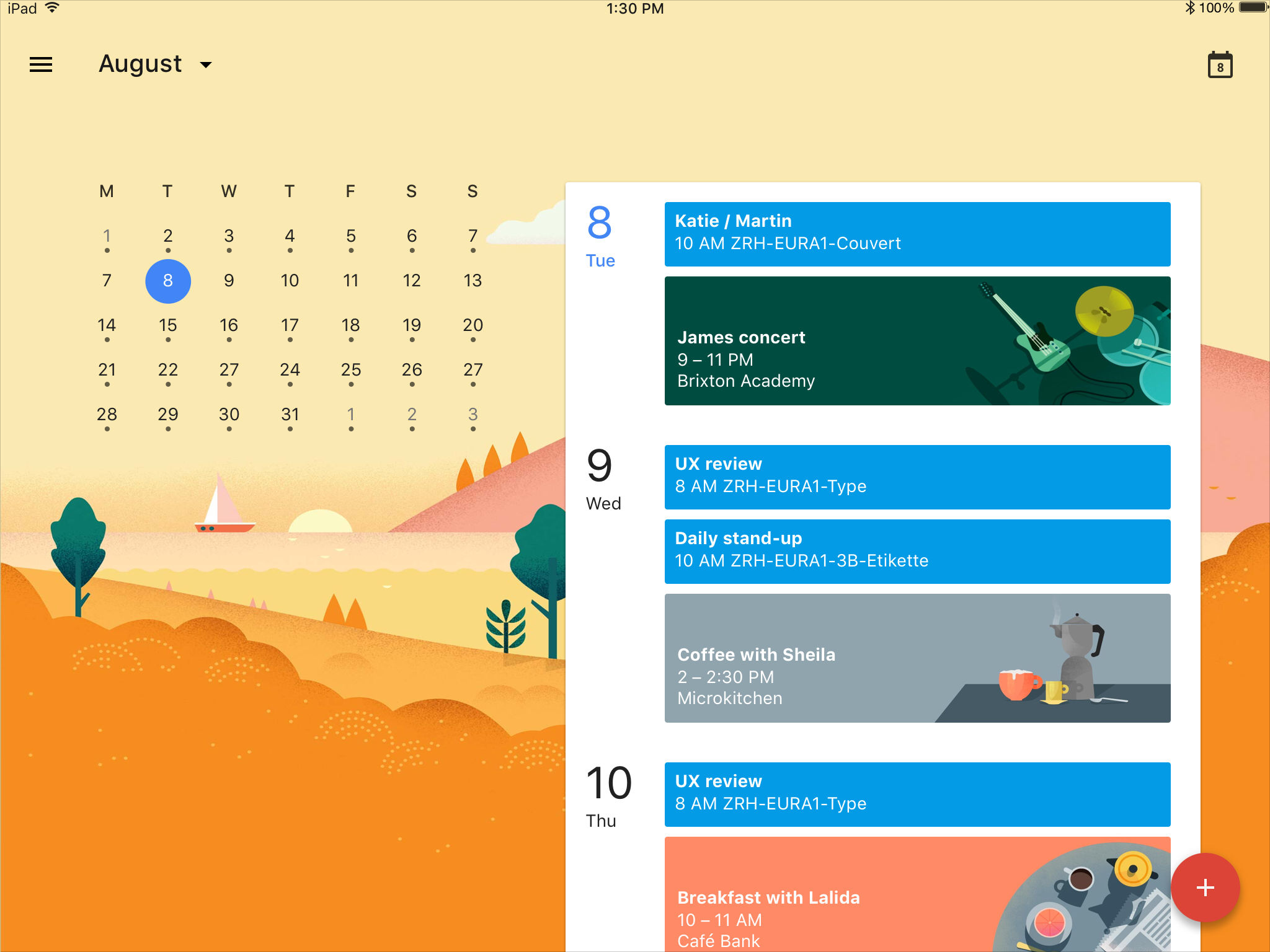Screenshot of an iPad's Home Screen Highlighting a Vibrant Calendar and Events

In this screenshot of an iPad’s home screen, the iPad’s interface details are clearly visible. At the top left corner, the "iPad" label is present, accompanied by the time displayed as 1:30 PM in the center top and the battery status at 100% in the top right corner. 

The left side of the screen features a detailed calendar for the month of August, indicated by the month’s name followed by three horizontal parallel bars, representing an interface menu. The calendar starts on a Monday, with the current date, the 8th, highlighted in a blue circle. This month spans from Monday, the 1st, to Thursday, the 31st.

The iPad's background is a whimsical and colorful landscape. This vibrant scenery features an orange sky with pink hues, stylized mountains, a calm sea hosting a small boat, a shining sun, and scattered trees that enhance the picturesque view.

To the right of the calendar, several upcoming events are listed:
- **August 8th, Tuesday**:
  - 10:00 AM: Katie/Martin meeting.
  - ZRH-EURA1: Kuvert.
- **August 9th, Wednesday**:
  - 9:00 - 11:00 PM: James concert at Brixton Academy.
  - 8:00 AM: UX review.
  - 10:00 AM: Daily stand-up, ZRH-EURA3B, Etiquette.
  - 2:00 - 3:00 PM: Coffee with Sheila at Micro Kitchen.
- **August 10th, Thursday**:
  - 8:00 AM: UX review.
  - 10:00 - 11:00 AM: Breakfast with Ali at Cafe Bank.

This descriptive caption provides a thorough overview of the visual elements and event details depicted in the screenshot.